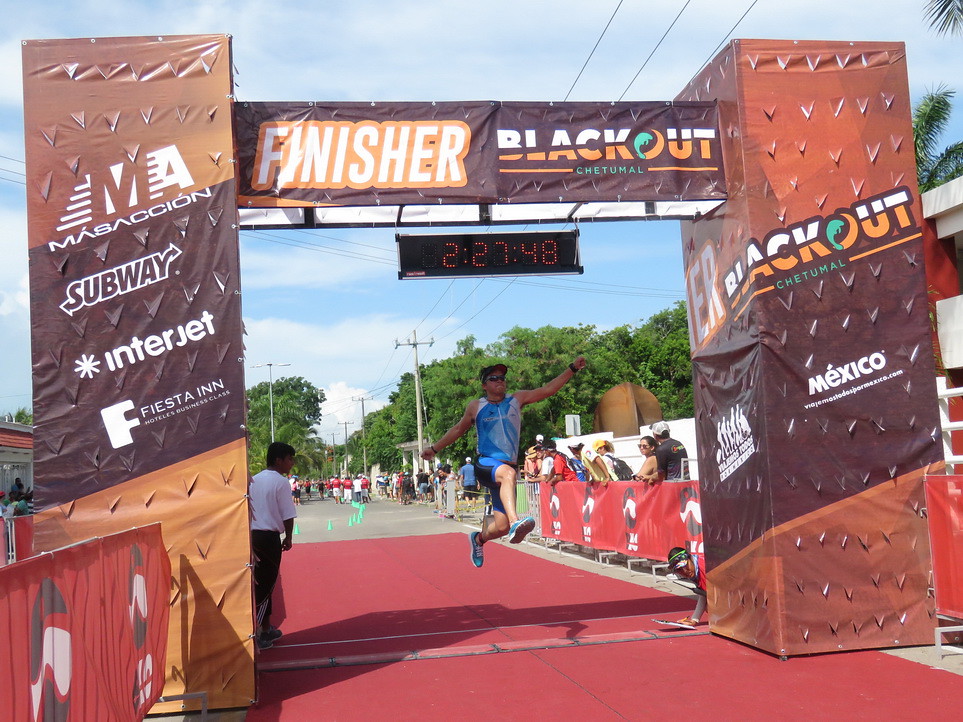The image captures the exhilarating moment at the finish line of a race, set against a bright, yet slightly cloudy, blue sky framed by tall, green-leaved trees. Dominating the foreground are two columns wrapped in material, supporting a banner proclaiming "Finisher Blackout Chetumal" (repeated on the sides), along with logos of sponsors including Subway, Interjet, Fiesta Inn, and a sign indicating Mexico. Mid-air at the finish line is a young man who has leaped triumphantly, wearing a blue sleeveless shirt, black and blue shorts, blue tennis shoes, and sunglasses. His dynamic pose shows one arm forward, the other behind, with legs stretched out as he crosses over a red carpet. His official finish time is displayed as 2:27:48. Nearby, behind a barrier, spectators watch the event, with a notable onlooker in a white t-shirt and black trousers observing the scene intently.